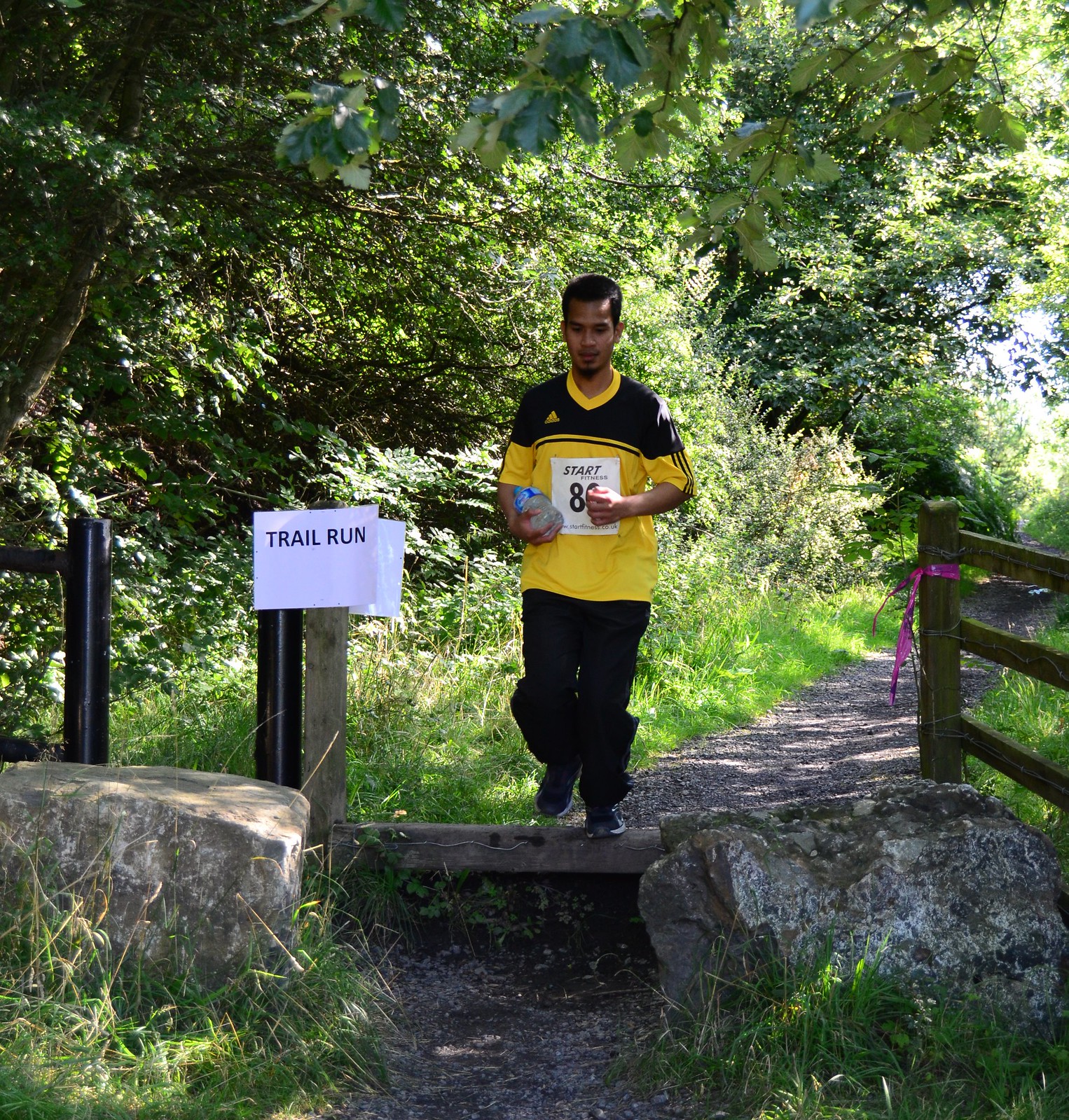This detailed photograph captures a young Hispanic man participating in a cross-country trail run. He is dressed in a yellow jersey with black shoulders and stripes, prominently displaying the number 80. The runner has short-cropped hair and a mustache and goatee. In his right hand, he clutches a bottle of water and exhibits an intense focus on his surroundings.

The trail he navigates is a narrow, gravel path winding through a lush, green forested area, possibly a city park. The path is lined with trees and grasses, providing ample greenery. To his left, a wooden fence runs alongside the trail, and to his right, the terrain dips into a rocky, ditch-like area. A white piece of paper with the words "Trail Run" is tacked to a post near him, marking the event. Additionally, a red bandana is tied to the fence post for further identification. The runner appears to be approaching a small set of stairs, poised to descend further along the trail.